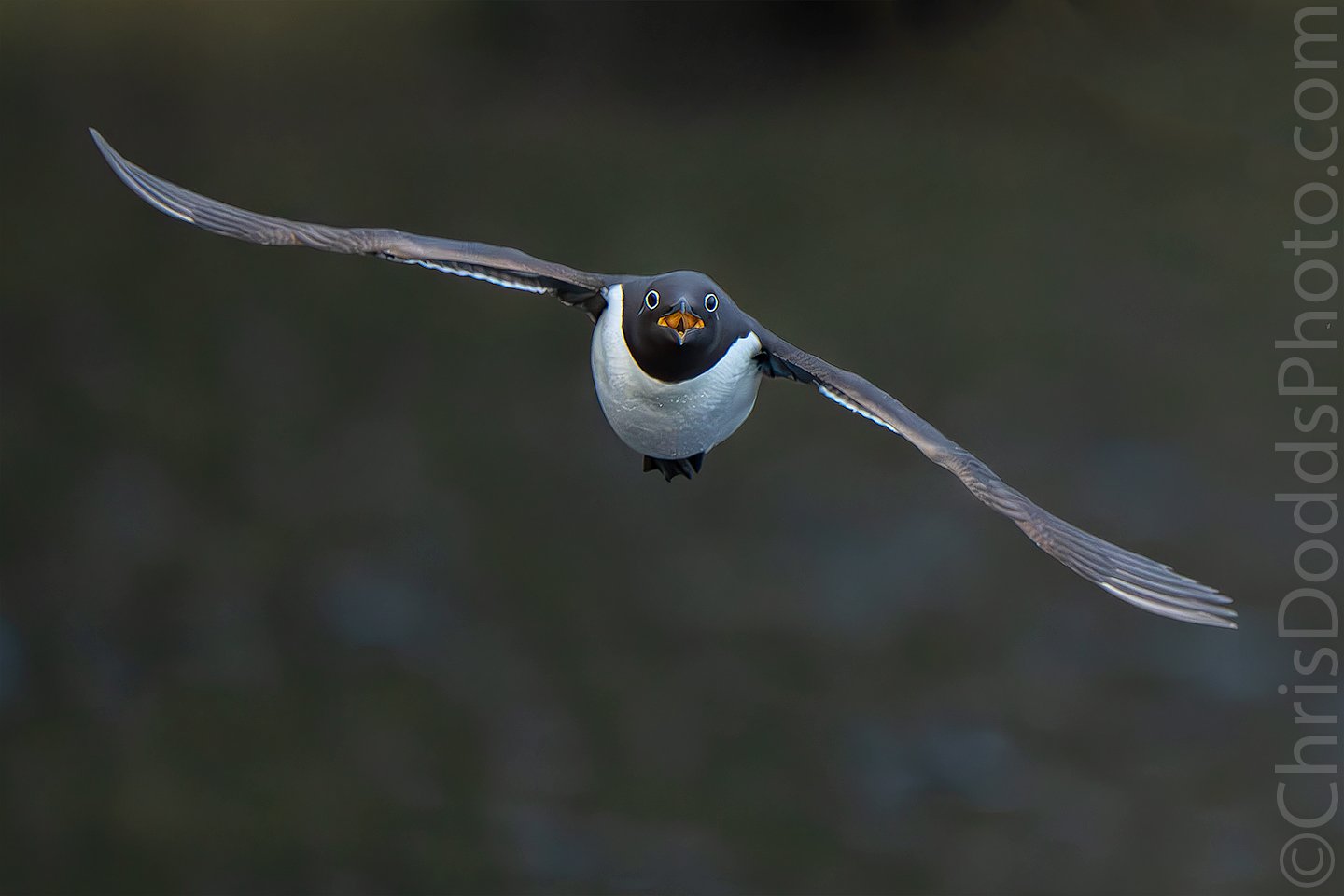This striking outdoor daylight photograph captures a bird in mid-flight, heading directly towards the camera. The bird, which has a nearly black head and neck, dark gray upper parts, and a pristine white belly, spreads its wings wide. The wings, predominantly white with dark edges, are held in a diagonal position, with the left wing higher than the right. Its black eyes, accentuated with a white ring, are fixed forward, giving an intense, almost comical expression. The bird's beak is open, revealing an orange-yellow inside, suggestive of it calling out. It also has small, black, webbed feet tucked underneath its body.

The background is dark and murky, likely portraying water or distant trees, which makes the bird stand out starkly in the frame. Along the right edge of the image, text reading "chrisdoddsphoto.com" accompanied by a copyright symbol, marks the image as the work of Chris Dodds. The overall effect is both dramatic and captivating, spotlighting the detailed plumage and expressive face of the bird.